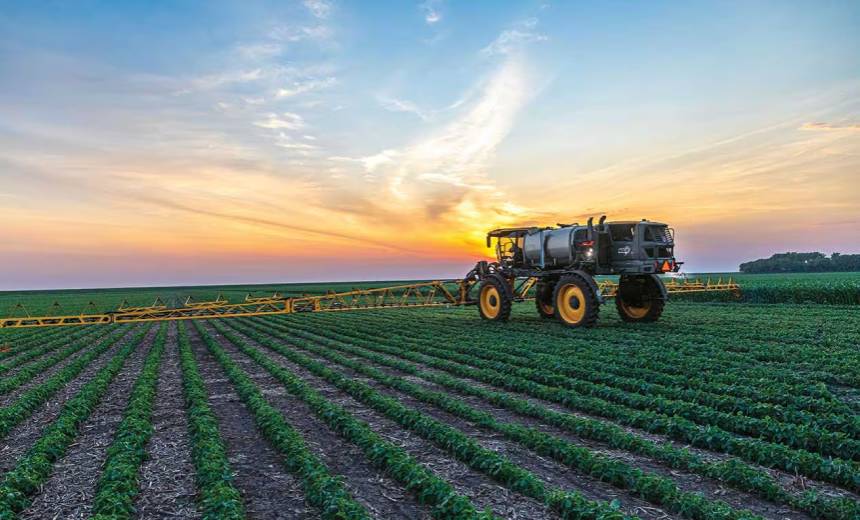The image depicts a vibrant farm scene, showcasing meticulously cultivated rows of green plants stretching out from the foreground to the horizon. The soil between the rows is a grayish-brown, creating a stark contrast with the vibrant greens of the plants. Prominently, a large yellow irrigation vehicle with oversized wheels is visible. The vehicle features extensive armatures that distribute water evenly over the crops and has a tank situated in its midsection. The vehicle's structure includes an elevated cabin at the front, and its design ensures that most of its body is elevated above its axles. In the middle distance, there's an orange safety sign, adding a splash of color. Beyond this, an area with taller plants can be seen, bordered by distant trees. The backdrop is a picturesque sky, transitioning from a warm orange at the edge – signaling the setting sun – to a cool blue as it extends upward.